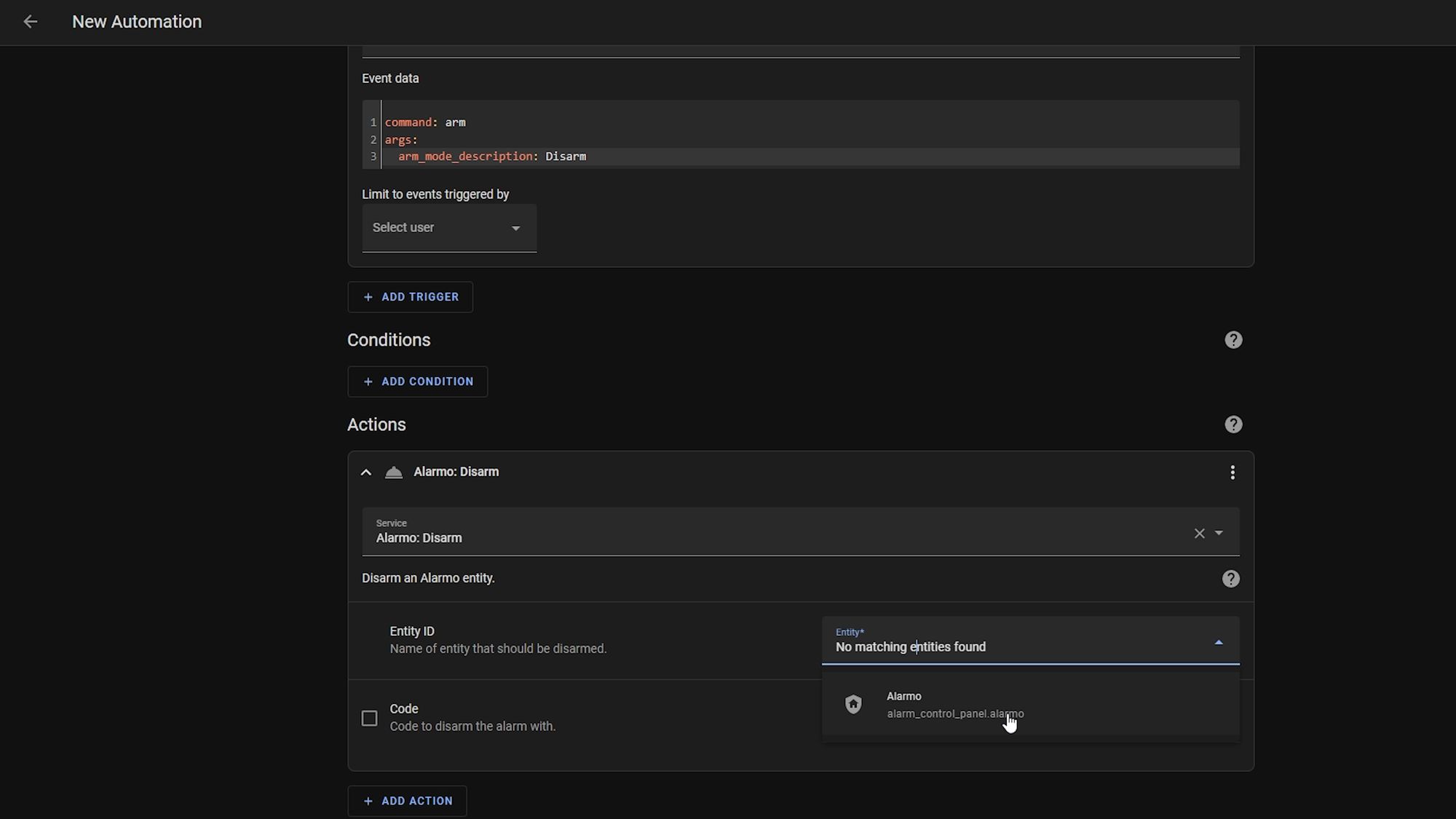The screenshot captures a computer screen with a predominantly black background, featuring text in white, blue, and orange colors. At the very top left corner, there is a black label that reads "New Automation" with a leftward-pointing arrow indicating the option to go back. Directly below this label, there appears to be small, possibly illegible text, which might say "Exact Data."

The majority of the screen displays distinct sections with different functionalities. Orange text highlights specific information beneath the hard-to-read smaller text. Below the orange text, a blue label titled "Add Trigger" is present.

Following this, there are two clearly marked sections. The first section, denoted with "Conditions" in larger white letters, includes an option labeled "Add Condition." The second section, similarly styled, is marked "Actions," with an underlying option that says "Add Action" in blue text located at the bottom left of the page.

In the lower part of the screen, within a black square containing additional smaller information, there is a smaller rectangle positioned at the bottom right. This smaller rectangle features a blue bar under its heading, with the heading itself presented in larger white font. This structured layout suggests that users can interact with and select various options to configure automation settings.